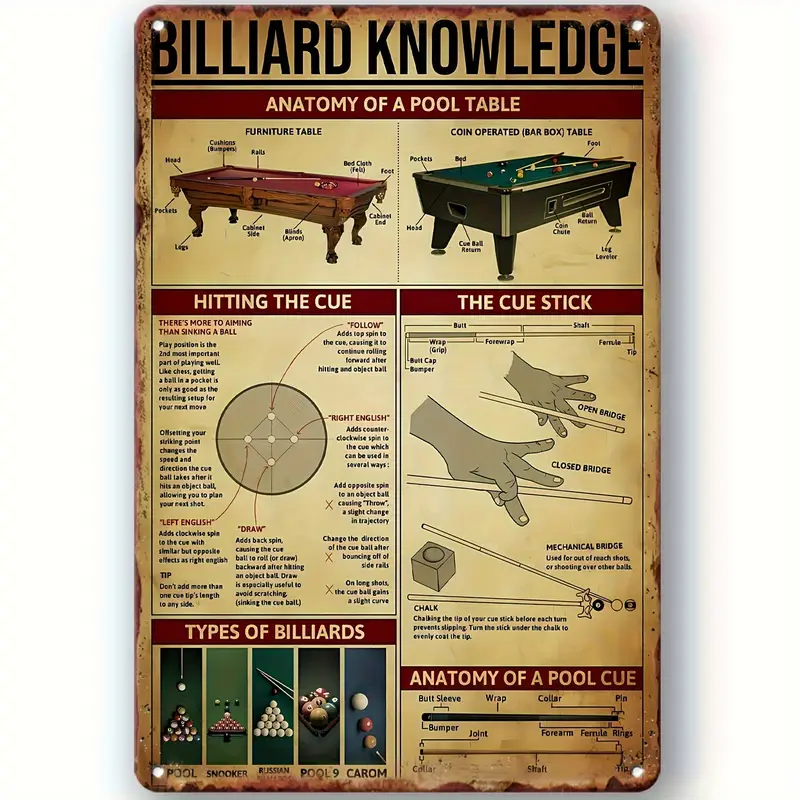The image is of an old-fashioned, ivory-colored metal sign with a weathered look, including rust around the edges and tiny holes in all four corners for hanging. The sign is titled "Billiard Knowledge" at the top in black lettering. Below this, the sign features a red background with the heading "Anatomy of a Pool Table." The sign is divided into several sections, each containing detailed illustrations and labels.

On the left side, the "Furniture Table" is depicted, showing everything labeled from the head and pockets to the feet and apron, with a red felt surface. To the right, the "Coin Operated Bar Box Table" is featured, with its own set of labels including foot, ball return, and coin shoot, highlighted by a green felt surface and metallic framing.

The middle left section titled "Hitting the Cue" offers tips on aiming and cue ball effects like "Left English" and "Follow," complete with diagrams. Adjacent to this, under "The Cue Stick," are illustrations showing different hand positions like Open Bridge and Closed Bridge, along with descriptions of the cue stick parts, such as the wrap, shaft, and ferrule. 

The bottom left corner elaborates on "Types of Billiards," with labeled images for various games like Pool, Snooker, Russian Pool, Pool Nine, and Carom. On the bottom right, the "Anatomy of a Pool Cue" is detailed with arrows pointing to the parts of the cue stick, from the butt cap to the bumper. The sign combines aesthetic appeal with comprehensive educational content on billiards.